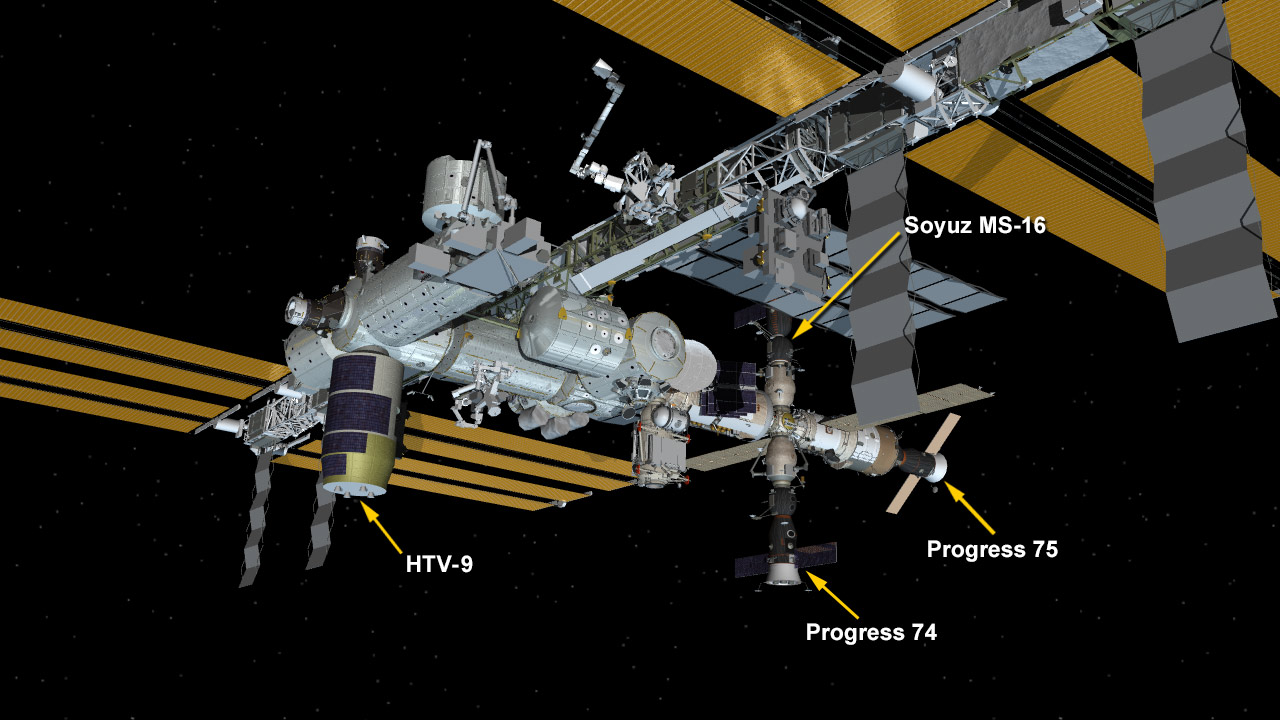This is a detailed, color computer-generated image depicting a satellite or space station in the vastness of space. The background is black, peppered with small white dots representing distant stars. The central figure is a predominantly silver, multi-cylindrical structure adorned with a variety of protruding components, including radar dishes, cameras, and telescopic instruments. This central cylindrical body is intersected by four elongated, metallic lines in a golden hue, likely representing solar panels, which extend horizontally.

Attached to the central structure are three space capsules, distinctly labeled with yellow arrows and white text: "Soyuz MS-16," "Progress 74," and "Progress 75." Another cylindrical section is labeled "HTV-9." The metallic space station, including these labeled sections, spreads from the middle left to the top right edge of the image. The various parts of the station and the attached objects underscore its complex and multifaceted nature, capturing the advanced technology required for space exploration. The color palette features primarily orange-gold, silver, metallic gray, light blue, and black hues, contributing to the image's technical and space-bound aesthetic.